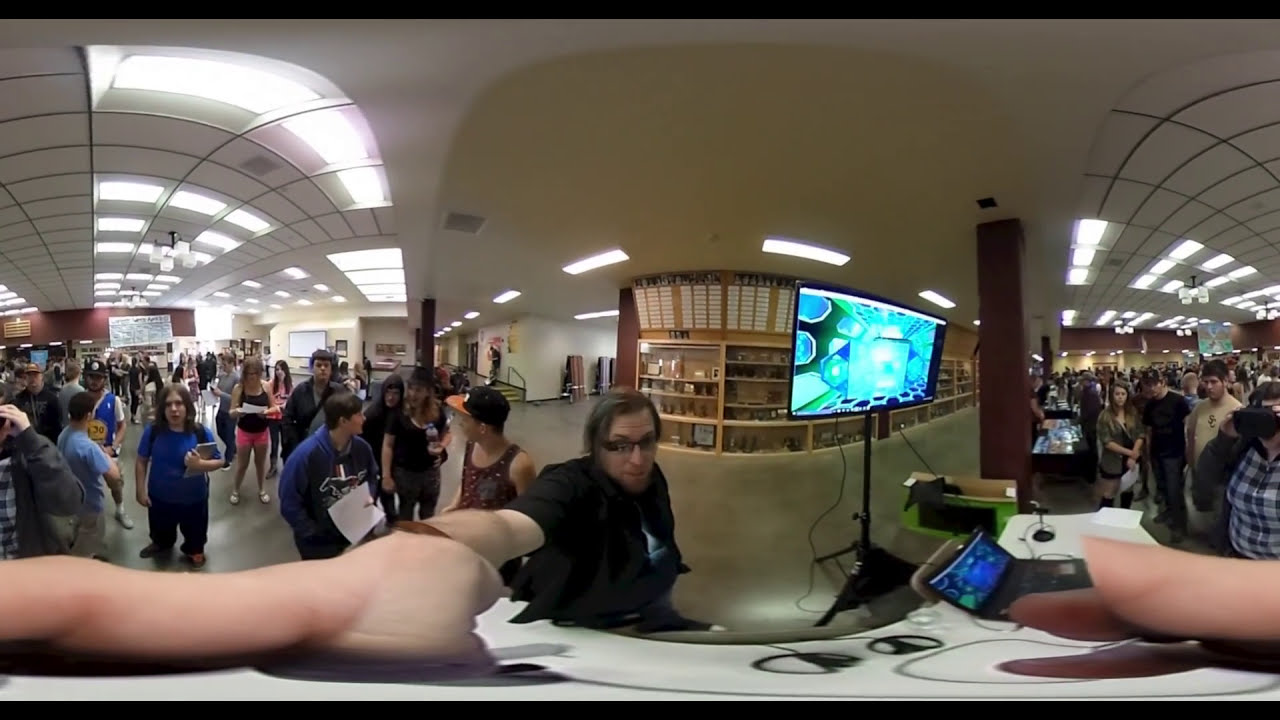In a large, bustling room with curved ceilings adorned with lights, a crowd of over 40 to 50 people stand in line, creating the effect of two hallways converging in a fisheye view. The individuals appear to be students, perhaps in a high school or college, dressed in various attire and holding books as they move towards several desks scattered around the room. At the center of the image, a white male with brown hair and dark glasses takes a selfie, extending his right arm to hold the camera. He wears a black shirt, and his visage is slightly distorted due to the panoramic lens. Directly behind him, attached to a black tripod, is a screen monitor. To his left, along the walls, glass display cases possibly filled with trophies and championship names add to the room's academic ambiance.